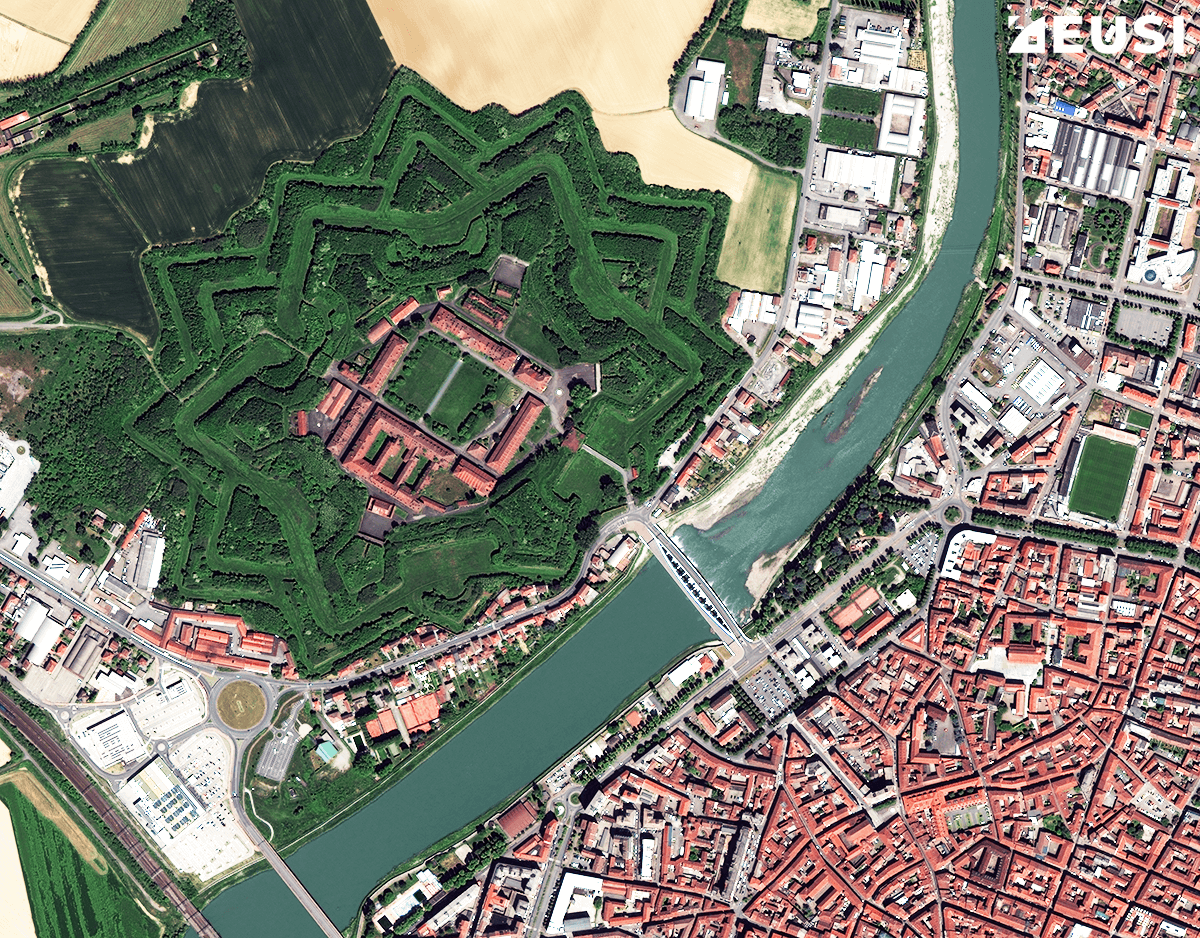This image is an aerial or highly detailed satellite view of a metropolitan city situated along a river. The river, featuring a striking sea foam green hue, meanders from the upper right to the lower left of the image, intersected by two notable bridges: a central white bridge and a further concrete bridge on the far left. To the right of the river lies a densely packed urban area with numerous buildings sporting terracotta roofs. The area is interwoven with various gray, blacktop roads. A prominent feature on the right side is a green field with visible line markers, likely a football field. On the left side of the river, open green spaces are more prevalent. One particularly striking landmark is a complex of buildings with terracotta roofs, surrounded by star-shaped landscaping composed of well-manicured shrubbery or trees. This combination of detailed natural and urban elements paints a vivid and intricate portrait of the city's geography and structure.